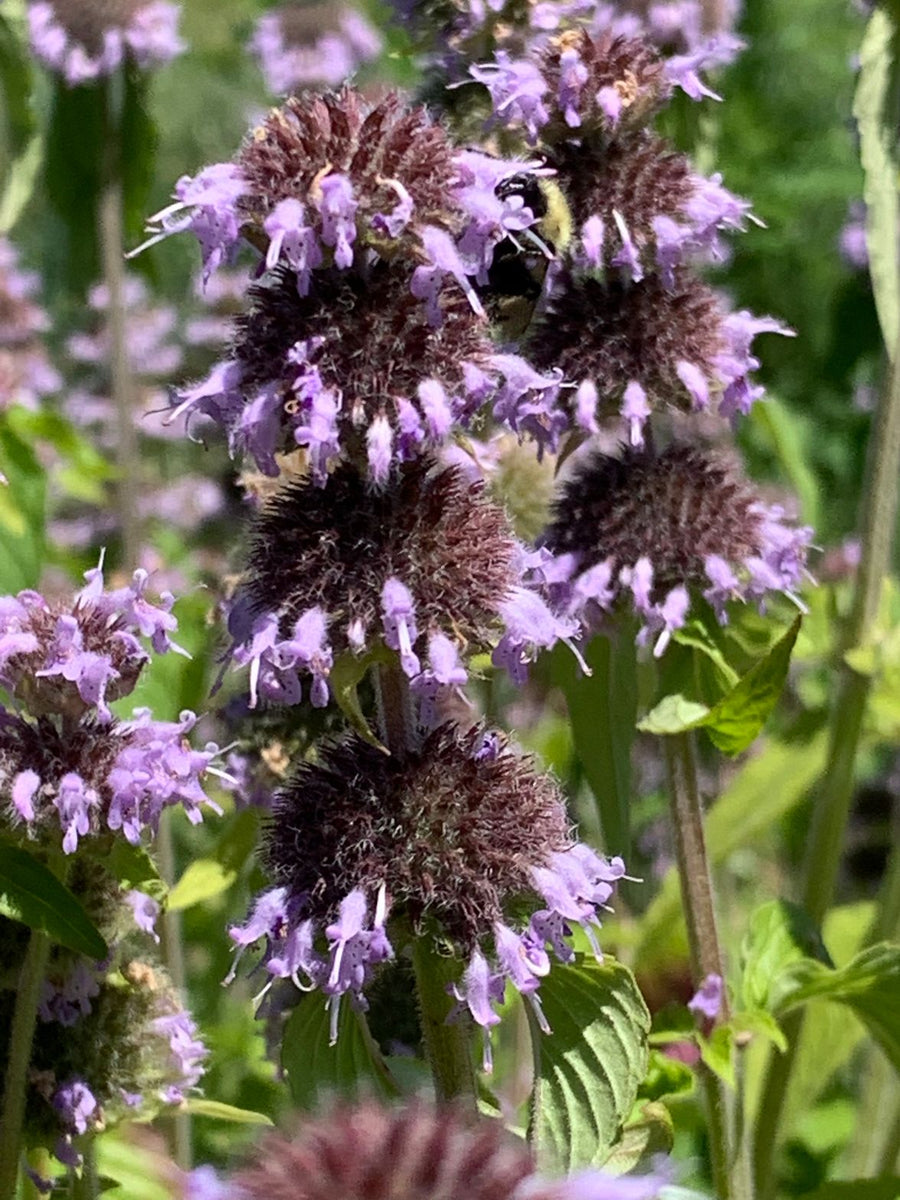This image showcases a close-up of several green-stemmed plants adorned with clusters of large, light purple, clover-like blossoms that appear past their prime. Each flower cluster resembles a stack of half-spheres with fuzzy, dark purple filaments emanating from them. The petals are fading and beginning to fall off, exposing some brownish bulbs at their centers. The stems beneath the blossoms are notably square-shaped and fuzzy, leading down to pointed leaves with prominently deep veins. The green leaves at the base are visible and contribute to the image's vibrant yet aging floral scene. The background is slightly blurred, revealing a field of similar plants stretching out, bathed in sunlight and casting a dappled play of shadows, emphasizing the purplish hue dominating the scene.